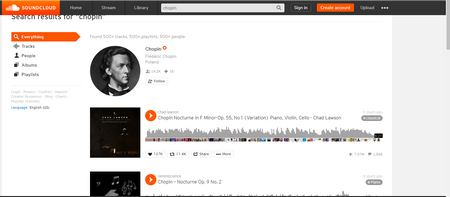The image depicts the SoundCloud interface open on a computer screen. On the left side of the interface, the distinctive SoundCloud logo, featuring a cloud icon, is prominently displayed. Below the logo, a vertical menu includes options such as 'Home,' 'Stream,' and 'Library,' with small icons next to each label. Above the main search bar, there are buttons for 'Sign In' and 'Create a Sound,' followed by another option that is partially obscured and unreadable.

The main content of the screen shows search results for the term "chopping." Underneath the search bar, filtering options are available, including 'Everything,' 'Tracks,' a partially legible 'Rare' option, and 'Playlists.' The search results include several tracks, with two discernible titles: "Chopping Nightmare Nighty" and "Chopping Nocturne." Each result is accompanied by a small cover icon, hinting at the audio content. The interface is neatly organized, allowing users to navigate and find content related to their search query efficiently.